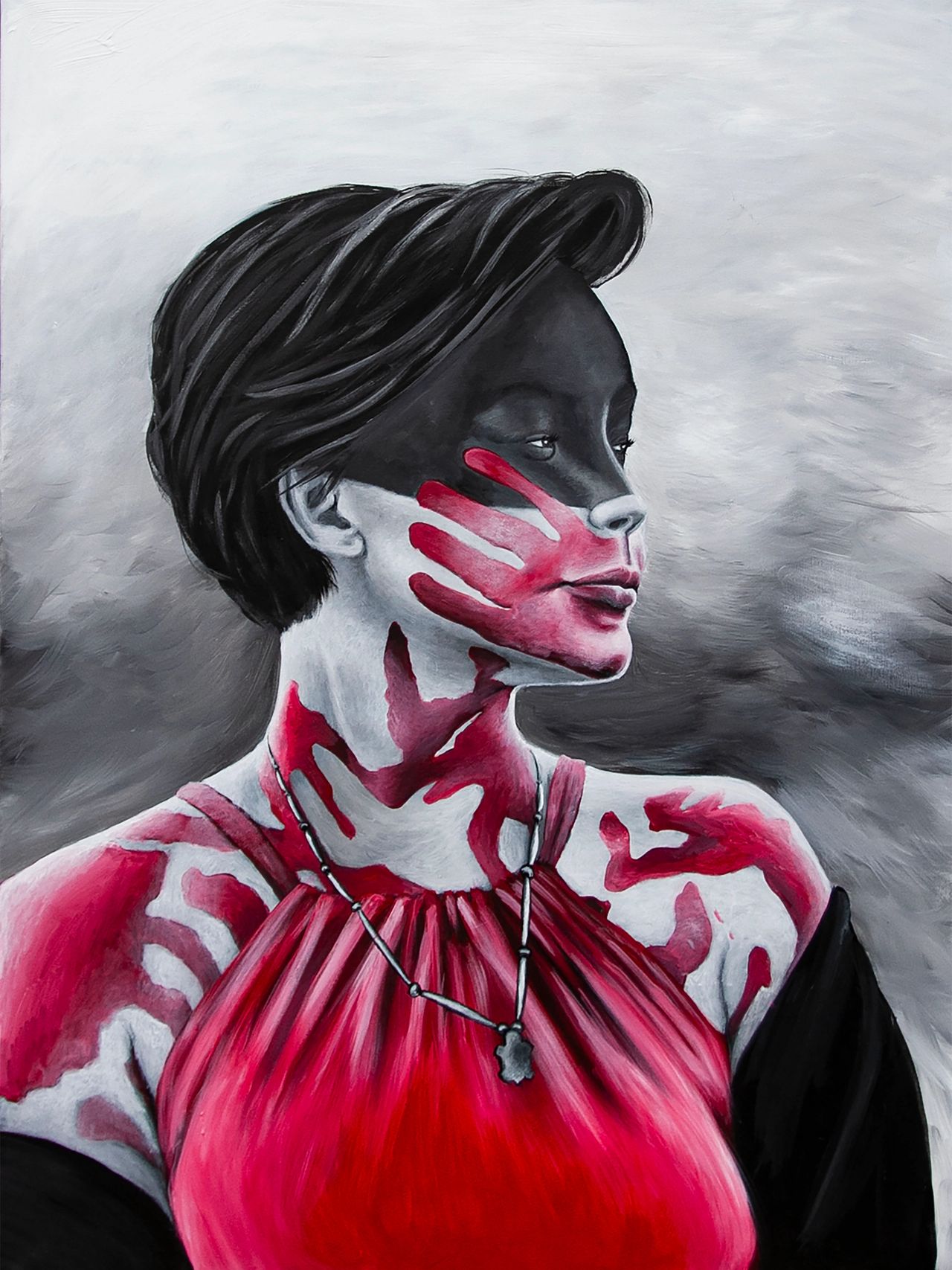This image is a detailed portrait painting, possibly hand-drawn or digitally created with a smooth animation style set against a swirling gray and white background. The central figure is a woman, likely in her 20s or 30s, with short black hair just below her ears, accented with gray streaks. Her face is strikingly painted: the top half is black, while the bottom half is white. A distinct red handprint spans from her lips to her right cheek. Further red markings, resembling abstract shapes or splatters, appear on her neck and shoulders, possibly suggesting paint rather than blood.

She wears a red halter-style blouse with thin straps around her neck, complemented by a silver necklace with a pendant that hangs to her chest. Over her lower arms, she drapes a black shawl or stole. The background features shades of gray, transitioning from lighter brush strokes at the top to darker tones near the center, framing the figure to draw attention to her detailed and symbolic visage.